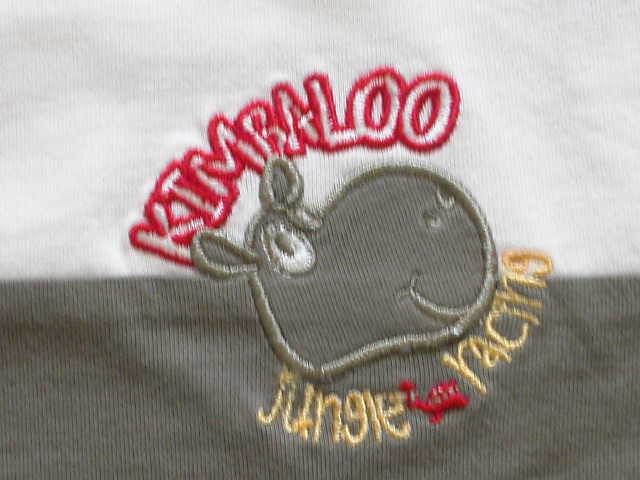This close-up image showcases a clothing item with a distinct two-tone design, featuring white on the top half and gray on the bottom half. Centrally positioned on the garment is an intricately sewn patch depicting a hippo's head. The hippo has large, expressive eyes with gray irises and white sclera, giving it a whimsical appearance. Above the embroidered hippo, the word "Kimbalo" is prominently displayed. Below the hippo's head are the words "Jungle Racing," separated by a small, red turtle-like emblem. The detailed stitching and vibrant colors make the design stand out against the fabric, creating a playful and eye-catching piece.